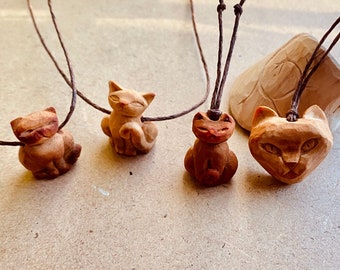This photograph captures a detailed arrangement of hand-carved cat figurines, which appear to be made of wood, displaying varying degrees of realism and charm. The scene features three full-body cat carvings, each attached to thin brown cords, suggesting they can be worn as necklace pendants. The cats are aligned side-by-side, each showcasing distinct characteristics: the first cat is chubby and somewhat flattened, the second resembles a Siamese cat, and the third features black ears with squinty eyes and a pink nose. To their right, there is a fourth carving of just a cat’s head, notable for its pointy ears and visible teeth, also attached to a brown string. In the background, resting on a light gray surface, lies another wood-carved object with subtle markings, adding a touch of artistic flair to the composition.